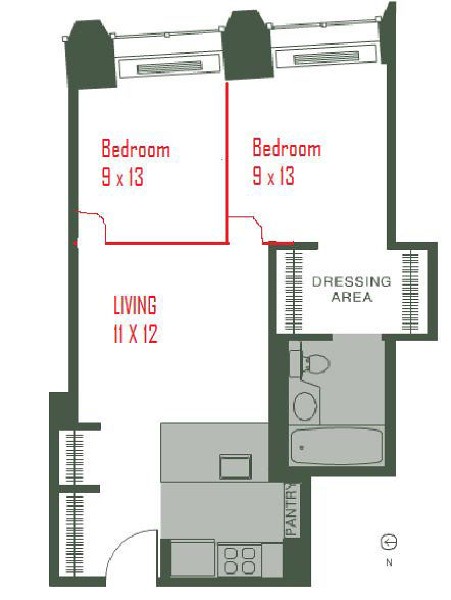The diagram illustrates the layout of a house or possibly an apartment, set against a white background with building outlines rendered in a deep hunter green shade. The various rooms are labeled with descriptive text, some in red for emphasis. In the upper-left corner of the image, there is a label in red indicating "Bedroom 9x13", with the room's lines also drawn in red. Adjacent to this on the right is another similarly labeled and outlined "Bedroom 9x13". Below the first bedroom, the text "Living 11x12" appears in red, indicating the living room area.

Adjacent to the second bedroom, and extending below it, the area is labeled "Dressing Area" in the same hunter green as the rest of the diagram. In the bottom-right corner of the image, a small black circle features an arrow pointing left, accompanied by a capital letter "N" positioned below it, likely denoting the northern direction.

Returning to the layout, a kitchen is situated below the living room space. Within the lower-right portion of the kitchen, a section labeled "Pantry" is marked vertically. At the top of the diagram, there are illustrations that could represent either shelves or window air conditioning units, located in both bedrooms. The detailed labeling and clear outline colors help distinguish each area within the living space.